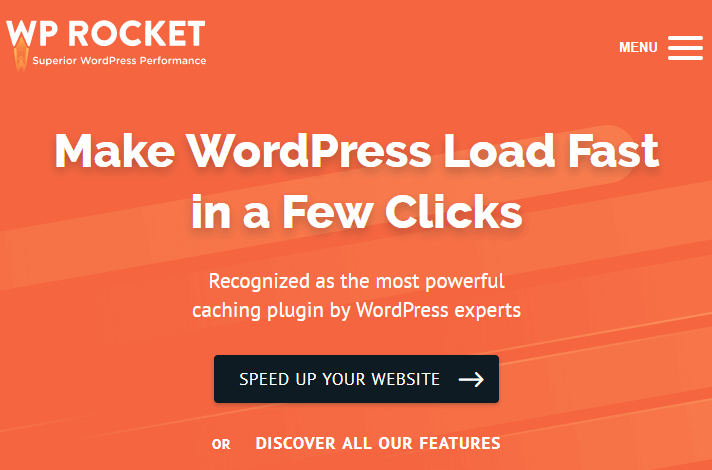The image appears to be an advertisement or a user interface screen for WP Rocket, a performance optimization plugin for WordPress. The background is solid orange, providing a vibrant and attention-grabbing backdrop. 

In the top left corner, there is a logo that reads "WP Rocket Superior WordPress Performance" in white text. The logo creatively incorporates a small trail of fire coming out of the 'W', resembling a rocket in motion, which reinforces the theme of speed and efficiency.

On the top right corner, there is a menu icon represented by three vertically stacked lines, commonly known as a hamburger menu, suggesting that this could be part of a software interface offering additional options.

Dominating the center of the image, bold large white text declares, "Make WordPress Load Fast in a Few Clicks," emphasizing the simplicity and effectiveness of the plugin. Below this, it mentions that WP Rocket is recognized as the most powerful caching plugin by WordPress experts.

The image concludes with a call to action in smaller white text: "Speed up your website" followed by "Discover all our features," suggesting two pathways for the viewer to engage with the product.

Overall, the combination of assertive text, branding elements, and navigation hints makes it likely that this image serves either as a promotional advertisement or as an introductory screen within the WP Rocket plugin interface.